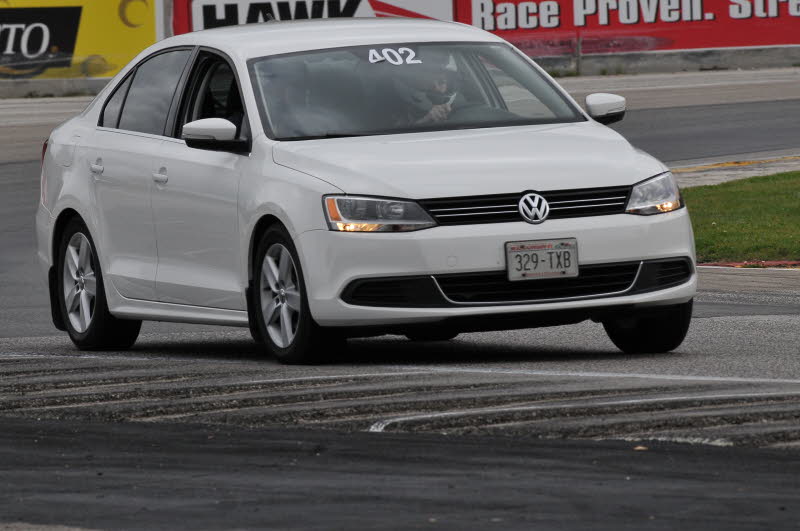The image features a white Volkswagen car on a racetrack resembling those used in NASCAR events. The racetrack, with its gray asphalt surface, has distinct white markings and a patch of grass in the center. The car, adorned with the number 402 on its windshield—where the number 4 is slightly peeling off—also sports a license plate reading "329 TXB." A driver, visible inside and wearing a helmet, can be seen gripping the steering wheel, with the car's lights turned on, specifically the parking lights, not the main headlights. Surrounding the racetrack are various advertisements, including a prominent yellow sign on the upper left and a red sign with white text saying "Hawk race proven" located from the middle to the right background. The scene is set during what appears to be dusk, adding a dynamic ambiance to the image.